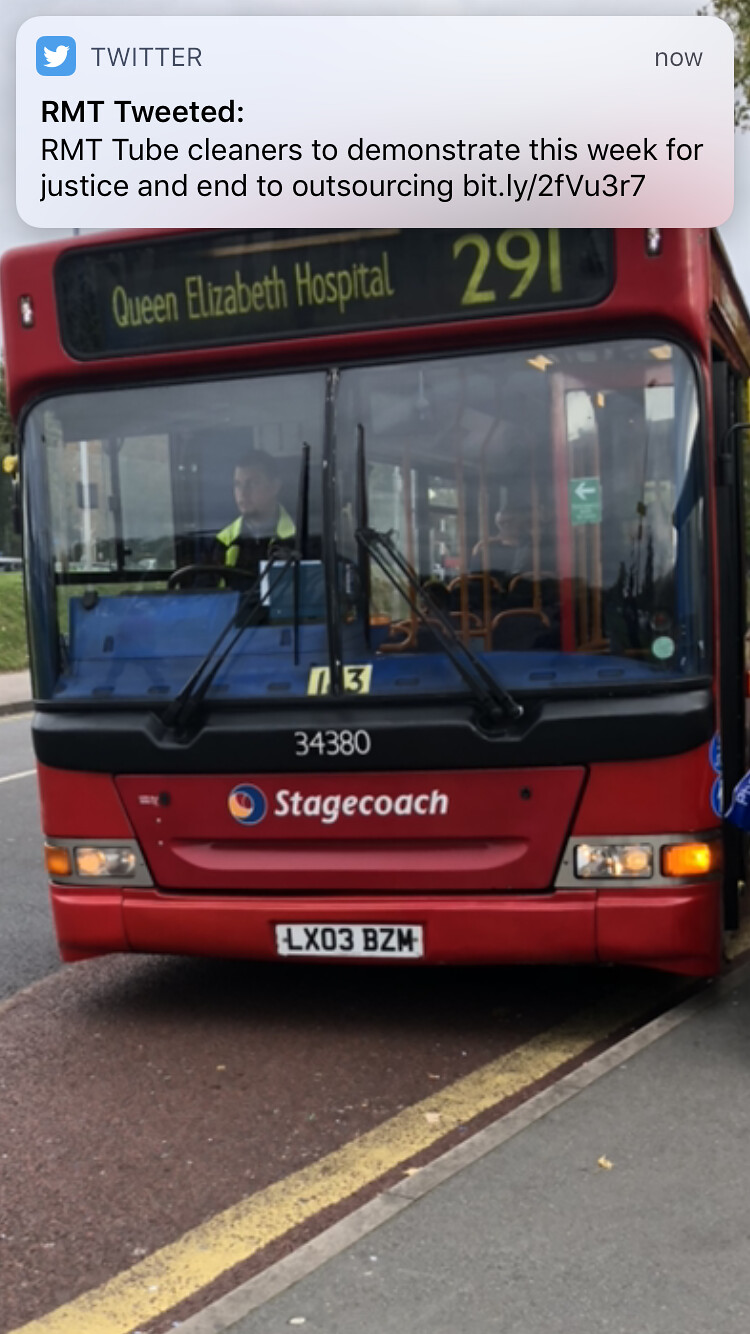The image is a horizontally-aligned, borderless screenshot that appears to be taken from Twitter, featuring a post by RMT about a demonstration. The top of the image includes the Twitter interface with the recognizable blue bird logo, "Twitter" in black, and "Now" on the far right. The tweet text reads: "RMT tweeted RMT tube cleaners to demonstrate this week for justice and an end to outsourcing bit.ly/2fvu3r7."

Beneath this text is a photograph of a red city bus prominently displayed in the center. The bus, primarily red with some black and yellow-green details, has a banner across the top that reads "Queen Elizabeth Hospital 291" in yellow-green letters on a black background. On each side of this banner, there's a small white spot against the red exterior of the bus. The driver's compartment, visible behind the glass, shows a blue dashboard, and various interior features include bars and poles for passenger use.

The driver, who appears to be a Latino male wearing a uniform with green or yellow epaulets and a blue shirt, is seated in the left-hand side of the bus. Black windshield wipers are visible below the driver’s window, and prominently displayed below this is the number "34380" in white letters. Further down, there is a horizontal red banner with the word "Stagecoach" in white capital letters, accompanied by a colorful logo to the left.

At the bottom-right side of the bus, various lights in orange, white, and yellow are present, with the orange lights positioned on the outer edges. The license plate reads "LX03 BZM." The bus appears to be parked near a gray sidewalk with a yellow line marking the boundary between the sidewalk and the street. The background suggests it is a sunny day, with visible grass beyond the bus.